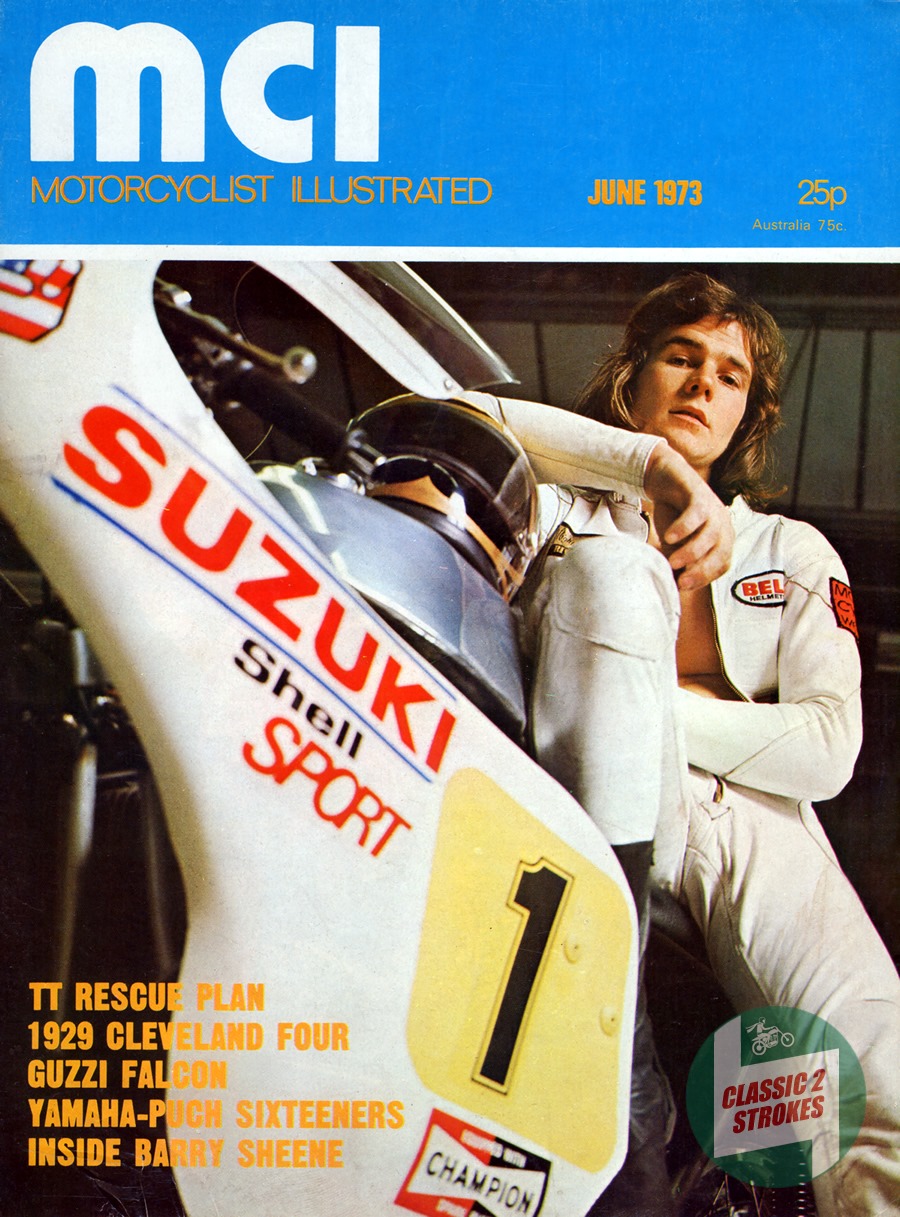The magazine cover features a detailed and vibrant image of a man lounging on top of a white racing motorcycle. The man, dressed in a slightly unzipped white racing suit, revealing a shirt underneath, has long brown hair and appears relaxed with his left leg perched on the bike and his right hand raised. A helmet rests underneath his right elbow on the motorcycle. The motorcycle prominently displays the name "Suzuki" in red letters along with a black number "1" set against a yellow background.

At the top fifth of the magazine cover, there is a blue banner with the magazine's title and issue details. In the top left corner of this blue section, "MCI" is written in bold white text, with "Motorcyclists Illustrated" in smaller yellow text beneath it. To the right, the banner reads "June 1973, 25P, Australia 75C".

The lower left corner of the cover is overlaid with yellow text detailing the magazine's features, including "TT Rescue Plan," "1929 Cleveland IV," "Guzzi Falcon," "Yamaha Puch 16ers," and "Inside Barry Sheen." Additionally, a round emblem in the bottom right corner highlights "Classic 2 Strokes." The cover masterfully combines the excitement of motor sports with the latest magazine content, making it an eye-catching presentation.